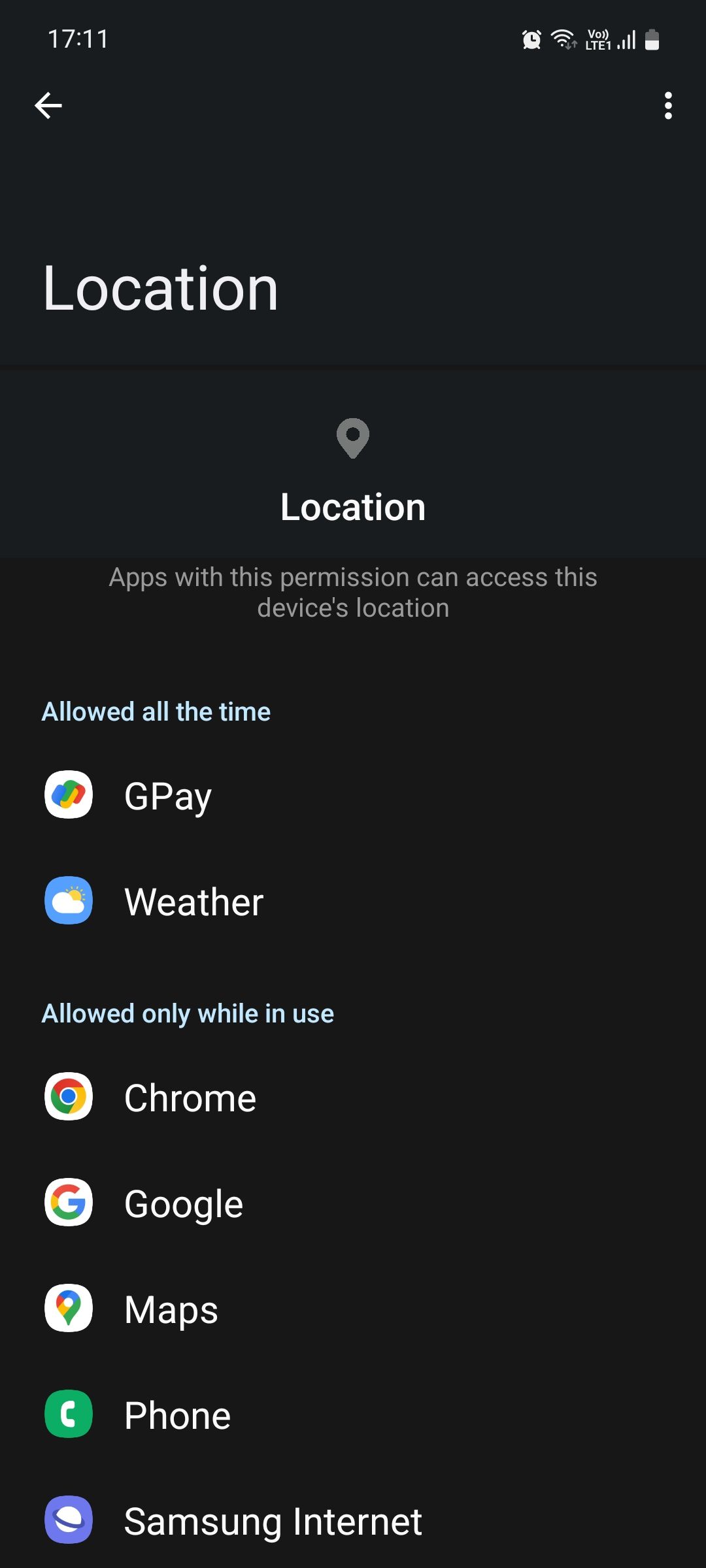This screenshot, captured from a cell phone, prominently displays the time "17:11" at the top along with an alarm clock icon indicating an active alarm, the Wi-Fi coverage indicator, and the battery status icon. Below that, the title "Location" is featured in bold text. The screen details the location permissions for various apps in white text on a black background. 

The section labeled "Apps with this permission can access this device's location" is followed by two lists. The first list, "Allowed all the time," includes:
- **GPay**: Represented by a white square with a blue, yellow, green, and red decorative element in the center.
- **Weather**: Shown as a blue icon featuring a white cloud with a yellow sun peeking from behind it.

The second list, "Allowed only while in use," includes:
- **Chrome**: Depicted as a circle made up of red, yellow, and green segments with a blue center.
- **Google**: An uppercase "G" made from segments of red, yellow, green, and blue.
- **Maps**: Shown as a directional icon with segments in red, blue, yellow, and green.
- **Phone**: Displayed as a green square with a white telephone handset.
- **Samsung Internet**: A blue icon featuring a white planet with a dark blue ring around it.

These icons are arranged vertically down the left side of the screen, providing a neat and organized list against the black background, making each app and its permissions easily identifiable.